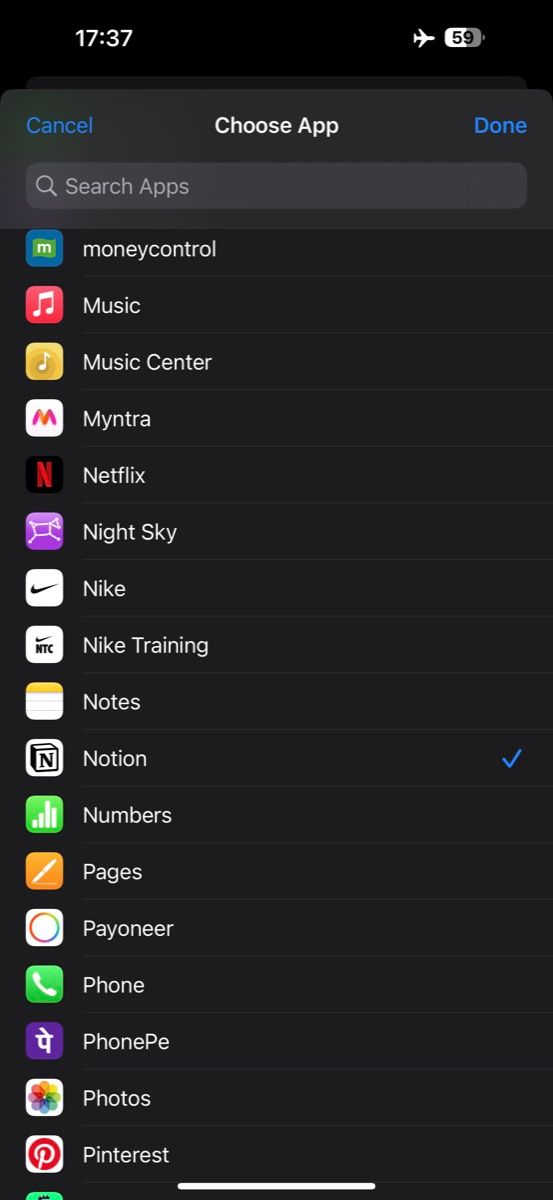In this image, a smartphone displaying an application selection screen is shown. The device is clearly an Apple product. At the top of the screen, the text "Choose App" is prominently displayed, with "Cancel" in blue on the left and "Done" also in blue on the right. Directly below, there is a search bar labeled "Search Apps."

The background of the entire image is black, providing a stark contrast to the list of apps below the search bar. The apps are listed vertically in the following order:

1. **Money Control** - Icon: Blue, green, and white.
2. **Music** - Icon: Red and white.
3. **Music Center** - Icon: Yellow and white.
4. **Mantra** - Icon: White and pink.
5. **Netflix** - Icon: Black and red.
6. **Night Sky** - Icon: Purple and white.
7. **Nike** - Icon: Black and white.
8. **Nike Training** - Icon: Black and white.
9. **Notes** - Icon: White and yellow.
10. **Notion** - Icon: Black and white with a black 'N' in a black box. This app is selected, indicated by a blue tick on the right side.
11. **Numbers** - Icon: Green and white.
12. **Pitches** - Icon: Brown and white.
13. **Pioneer** - Icon: White with a green circle.
14. **Colors** - Icon: Green, blue, orange, and yellow.
15. **Font** - Icon: Green and white.
16. **Font PE** - Icon: Purple and white.
17. **Photos** - Icon: White with a multi-colored circle (yellow, green, blue, red).
18. **Pinterest** - Icon: White and red.

Each app is easily identifiable through its distinctive icon, collectively providing a rich palette of colors against the black background.